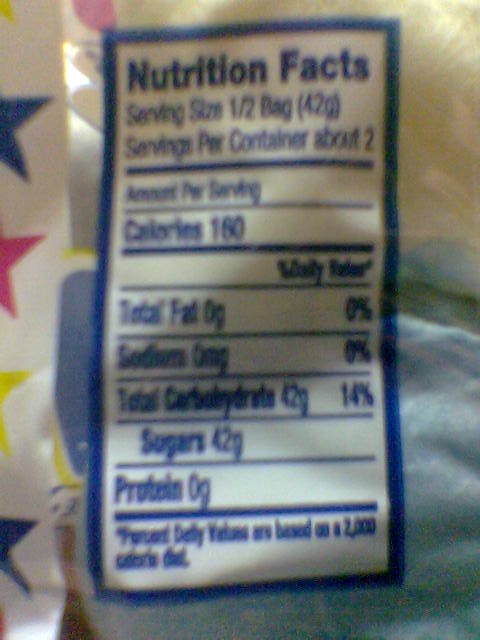The image showcases a packaged product prominently featuring nutritional information. The nutrition facts are displayed in a white rectangular box bordered in blue, with "Nutrition Facts" clearly labeled at the top in blue text. The packaging itself consists of a mix of clear and white plastic, allowing partial visibility of the contents inside. Around the white box with the nutrition facts, there's a hint of a yellow, red, and blue star pattern, adding a colorful touch to the otherwise plain background.

The upper portion of the plastic bag is mostly translucent, giving us a glimpse of a possible red circle behind the packaging, which seems to bleed through the material. The lower part of the package also shows the blue and white design elements partially visible behind the plastic. However, the exact contents of the package remain unidentified as there is no text or imagery indicating what the product inside might be.